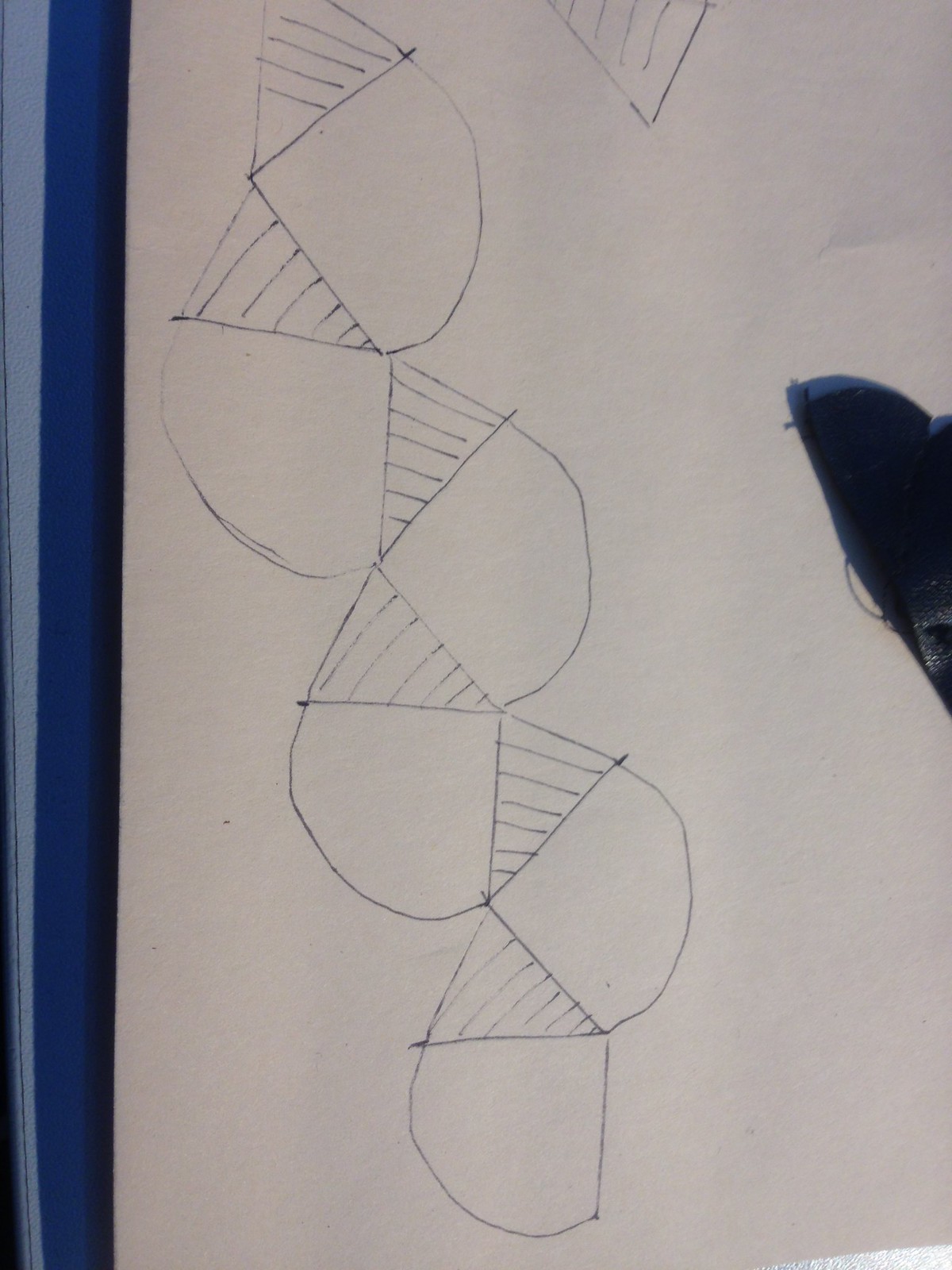This vertical portrait image predominantly features a color palette of blue, white, and black, reminiscent of a ballpoint pen line drawing. On the right middle edge, a dark spot shaped like a half dome draws the eye. The left edge is defined by a thick blue line, complemented by a thinner light blue line at the very boundary. 

At the center of the image, intricate pen line drawings capture attention. At the top edge, an inverted triangle with four horizontal lines connects seamlessly to a downward triangle adorned with vertical lines, creating a symmetrical pattern. An arc on the right connects the outer points of these triangles, establishing a harmonious design. This specific pattern of triangles and connecting arcs repeats two more times, cascading down towards the bottom edge, creating a visually engaging, continuous motif.